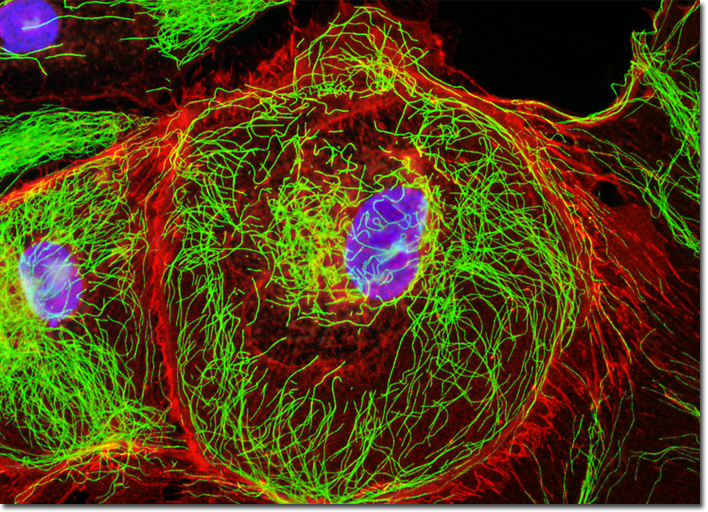This image presents a visually captivating and colorful composition, reminiscent of either an abstract art piece or a scientific microscopic image. It features a dark black background that dramatically highlights the intricate patterns in the foreground. Dominating the scene are vibrant neon green squiggly lines and threads, intertwined with intense reddish hues, creating a chaotic yet fascinating mesh. Scattered across this tapestry are three distinct purple blobs, each resembling a nucleus within an amoeba, adding focal points to the visual chaos. These purple areas slightly alter the color of the underlying green lines to white, contributing to the dynamic interplay of colors. The overall impression is one of a complex, possibly digitally created artwork, filled with energetic lines and colorful nuclei-like formations that evoke the appearance of microscopic life forms.